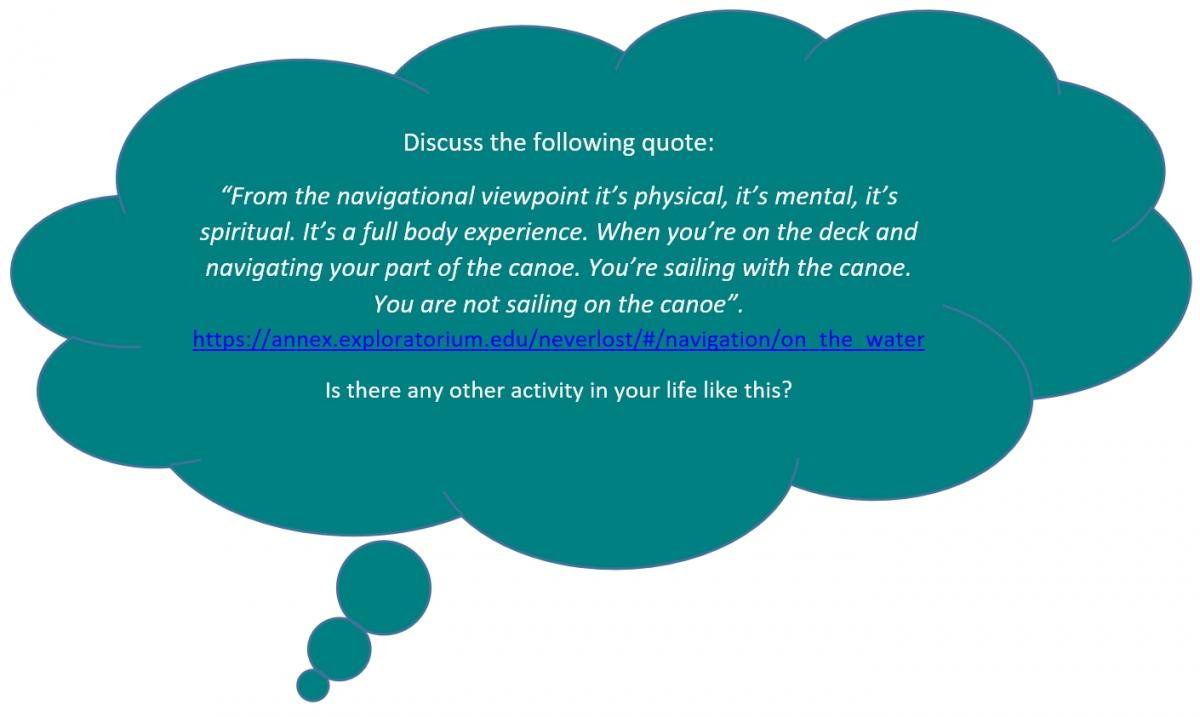The image features a large, green thought bubble occupying the entire frame. Inside the thought bubble, three dots trail downwards to the left, similar to the style seen in comic strips to indicate someone speaking. The bubble contains white text that reads, "Discuss the following quote: 'From the navigational viewpoint, it's physical, it's mental, it's spiritual, it's a full-body experience. When you're on the deck and navigating your part of the canoe, you're sailing with the canoe; you're not sailing on the canoe.'" A dark blue hyperlink, which is difficult to read and seems to say "annexexploration.edu," follows the quote. Beneath the hyperlink, another question in white text asks, "Is there any other activity in your life like this?" The context suggests the image may be a slide from a presentation or a prompt for a learning activity.